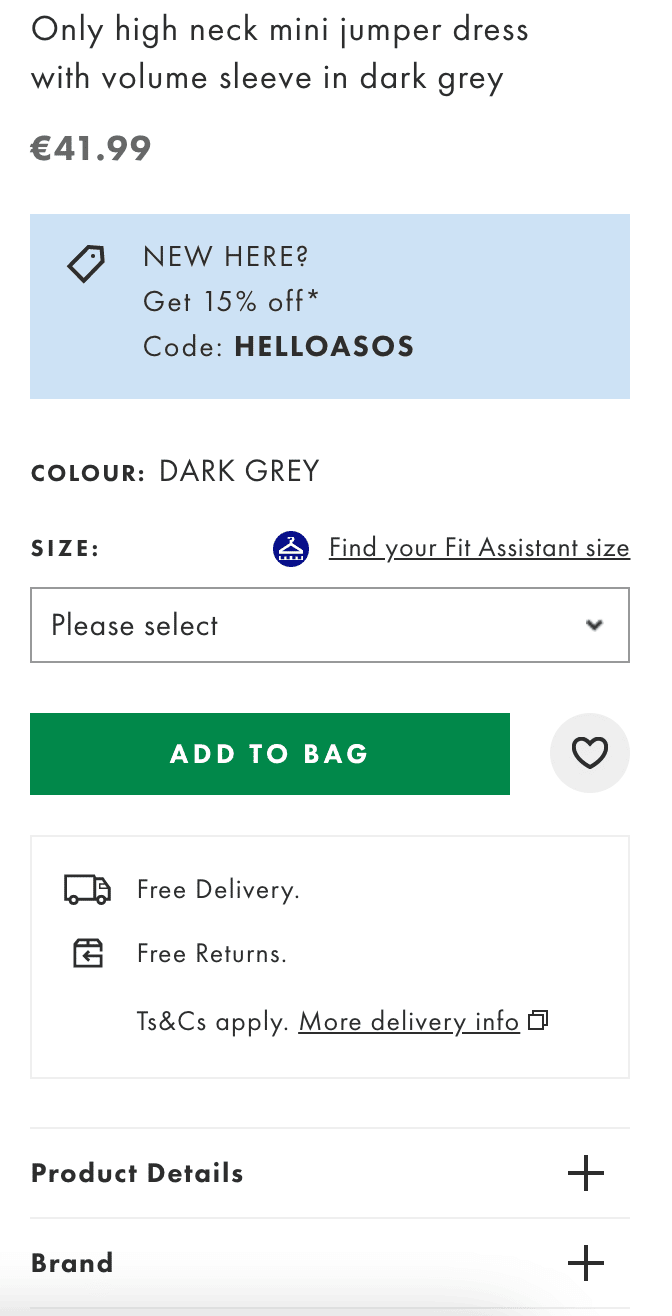**Descriptive Caption:**

This screenshot depicts the shopping page of a fashion website, showcasing a product titled "Only High-Neck Mini Jumper Dress with Volume Sleeve in Dark Gray." The dress is priced at €41.99. 

At the top of the page, a promotional blue box offers new customers 15% off their purchase with the coupon code "HELLOASOS." Directly below, the color option is highlighted as 'Dark Gray,' and the size selection remains unspecified. Another feature is a blue circular icon containing a hanger with beads, labeled "Find Your Fit - Assistant Size."

A prominent green rectangle button invites users to "Add to Bag." Below this call-to-action, it mentions benefits such as "Free Delivery & Free Returns" with a note indicating that terms and conditions apply (T&Cs). For additional shipping details, there's an underlined link saying "More Delivery Info."

Finally, sections titled "Product Details" and "Brand" are available for users seeking further information about the item.